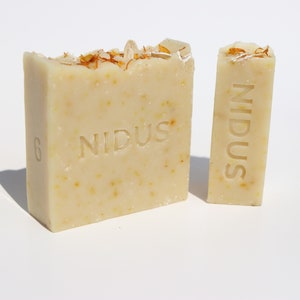The photograph showcases two irregularly cut soap bars in a cream-yellow-cheese color. Both bars prominently feature the brand name "Nidus" engraved on their surfaces, with the thicker and wider bar also displaying the number "6" on its left side. The narrower bar has the brand name "Nidus" inscribed vertically. The tops of both bars are rough and jagged, suggesting they were broken or cut. Inside the soap, there appear to be embedded decorative elements, resembling orange leaves or string-like materials, which are peeking out from the rough surfaces. The left bar, which is significantly wider and thicker, contrasts with the more compact, travel-sized right bar.